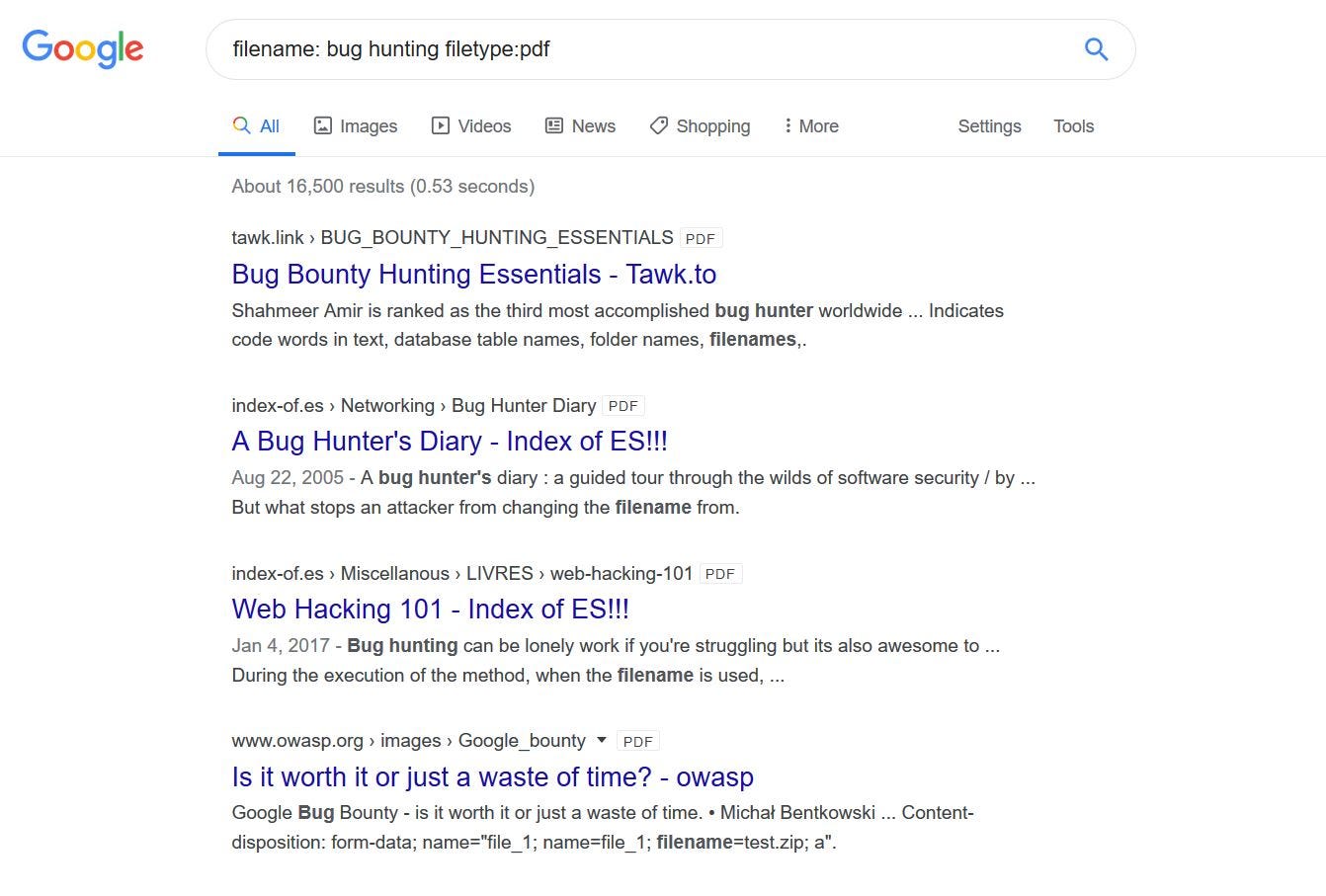The image depicts a screenshot of the Google website on a desktop screen. The page is set against a clean, white background. Prominently displayed at the top is the iconic Google logo. Below the logo, a search bar is clearly visible, containing the text "file name: bug hunting, file types: PDF" in black font. To the right of the text is the recognizable search icon.

Beneath the search bar, a navigation bar offers various categories for search results, including "All," "Images," "Videos," "News," "Shopping," and "More." The label "All" is highlighted in blue ink and is underlined with a blue line, indicating the selected category. Further right, the options "Settings" and "Tools" are presented in a subtle gray ink.

The search results section follows, beginning with a small text line that reads "About 6,500 results (0.53 seconds)" in gray ink. The results themselves feature headings in blue ink, each one serving as a clickable link to external websites. The first result is titled "Bug Bounty Hunting Essentials," followed by "A Bug Hunter's Diary," "Index of ES," and "Web Hacking 101." Another result reads "Is it worth it or just a waste of time?" Each of these headings is accompanied by a short description in dark gray or black font, providing brief summaries of the content behind the links.